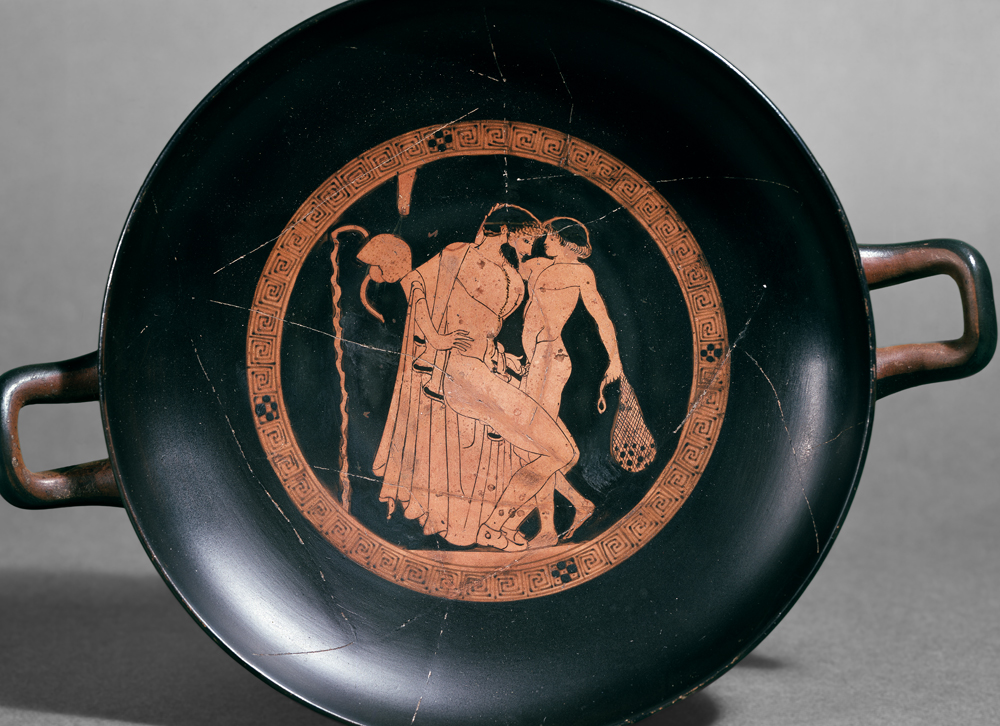This image features a circular Greek-style decorative plate or pan with an ornate, black, and orange design, standing upright. The plate has two dark cherry wood-colored handles on each side, suitable for gripping with two fingers. In the center of the plate, there is an intricate depiction of an ancient scene rendered in a distinguished 2D flat style reminiscent of classic Greek pottery. The scene portrays a larger man on the left wearing a cloak and possibly a soldier's helmet and holding a cane. He is reaching out with his left hand towards a smaller, fully naked young boy on the right, who is also depicted holding a netted bag. The larger man has visible genitalia, with an erect penis, while he appears to be gripping the smaller man's non-erect penis. The overall artwork seems to present a controversial, intimate moment between the two figures, captured in the detailed and aged aesthetic typical of historical Greek art.